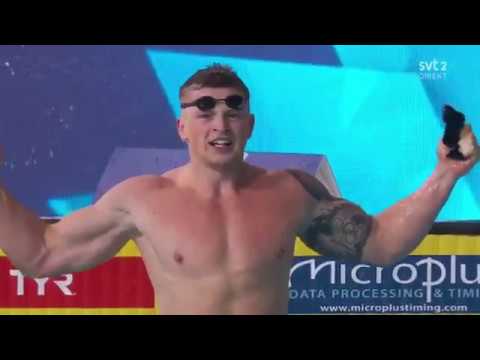A muscular swimmer in his mid-30s, standing shirtless with his arms raised, showcasing a large, dark tattoo on his left shoulder. His well-defined physique and perfect form suggest he is at the peak of his athletic career. He wears black swimming goggles, positioned above his eyes and strapped securely to his forehead. In his left hand, he holds an indistinct black object. The background features a pattern of turquoise blue rhombuses, contrasting with his fit and focused appearance. His pinkish-brown nipples and chiseled muscles add to the details of the image.